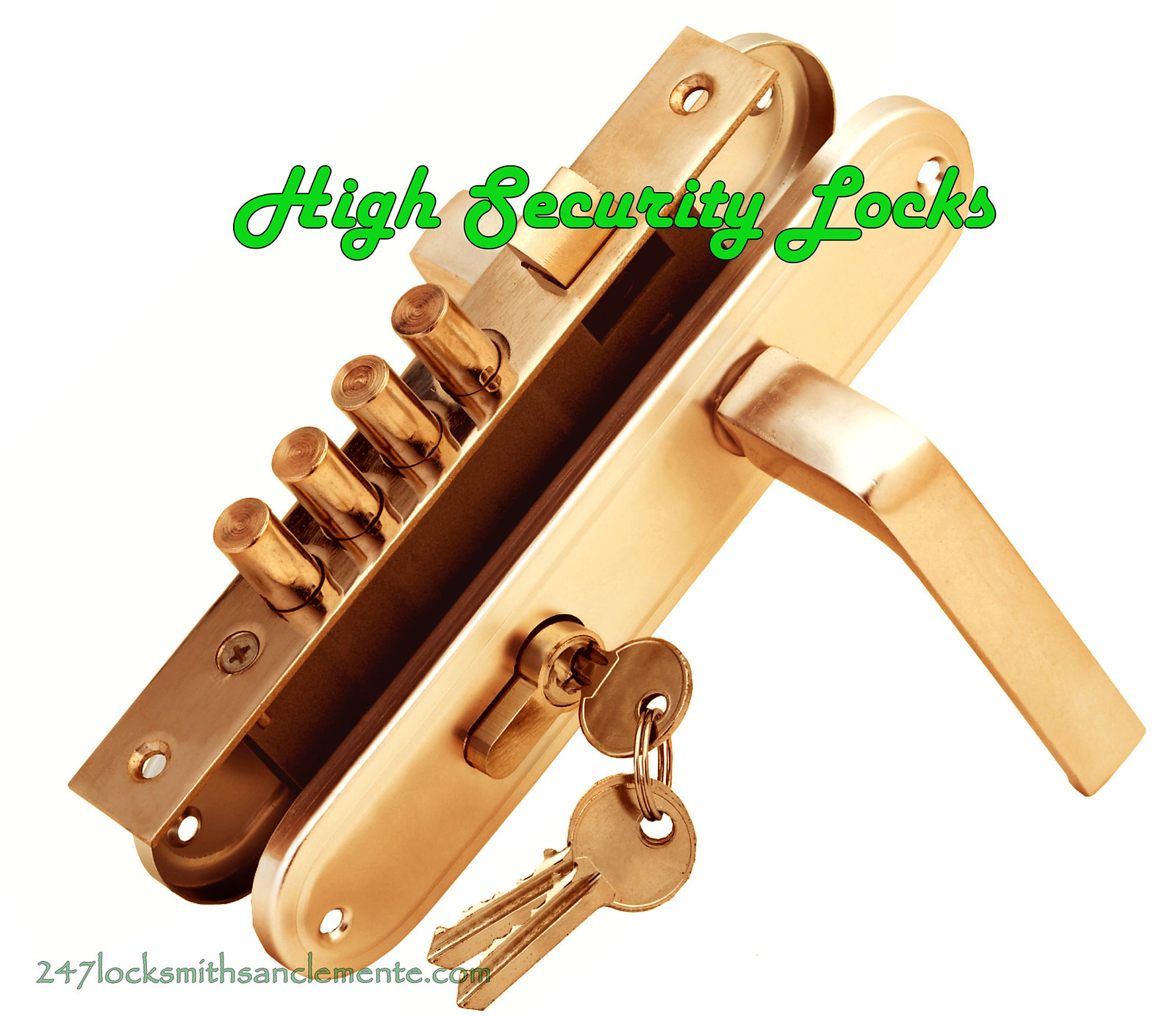The image appears to be an advertisement for a high-security door lock, prominently featuring a dismantled brass lock mechanism set against a pure white backdrop. The lock, oblong and rectangular, showcases a side lever-style handle that juts out in an L-shape, designed for a downward push. Directly beneath the handle, a small round key is inserted into the keyhole, attached to a keyring with two identical keys dangling from it. The brass lock mechanism includes four protruding cylinders and an additional handle visible on the opposite side, hinting at a comprehensive locking system. Diagonally aligned from the lower left to the upper right corner, the product is captioned at the top with "High Security Locks" in stylish bright green cursive lettering. The bottom left corner features a slightly translucent silver text that reads "24-7 Locksmith, SanClemente.com," adding a professional touch to the advertisement.